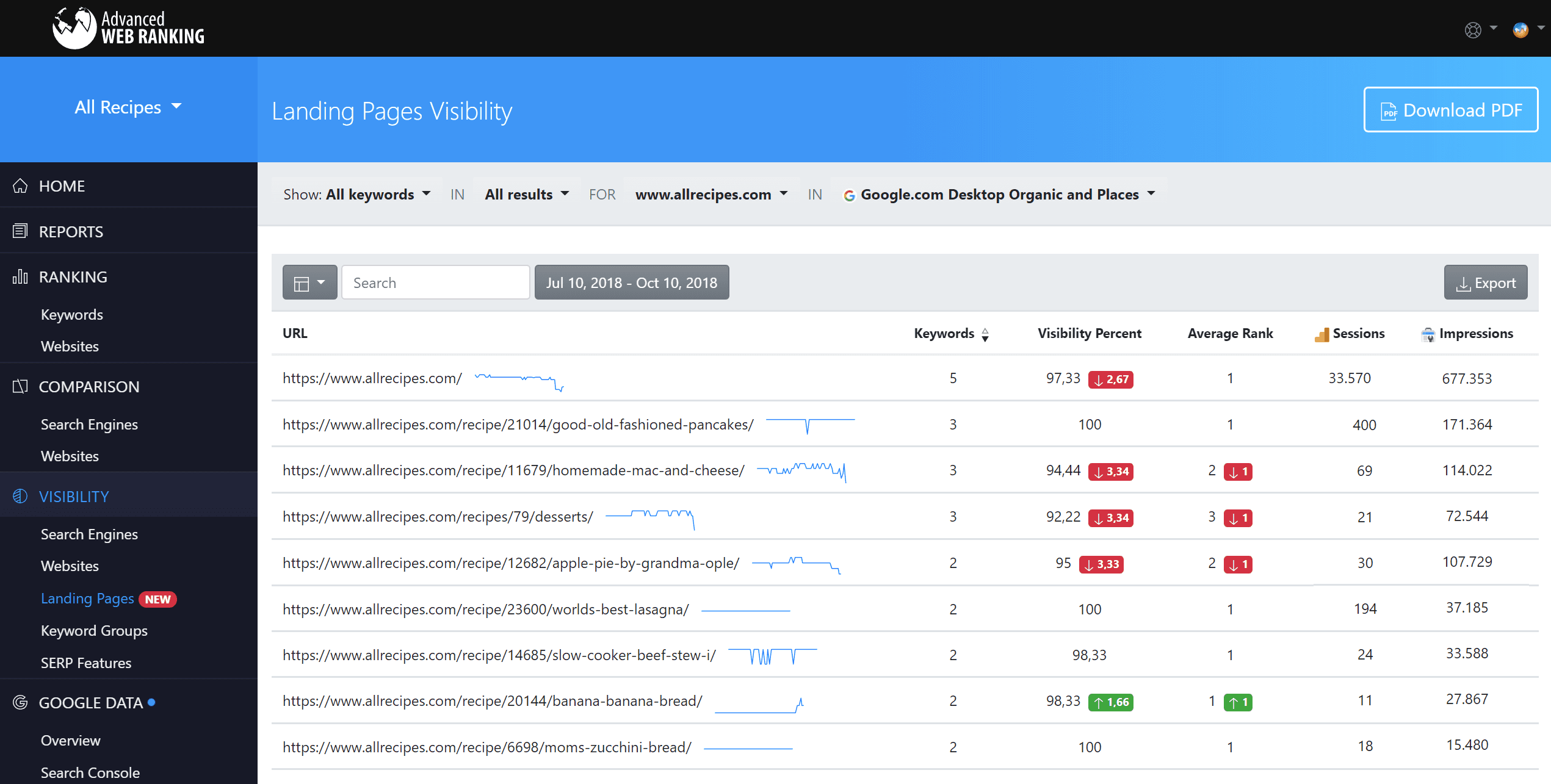This screenshot features a detailed view of the Advanced Web Ranking platform on a laptop screen, located in the upper left-hand corner. A small, white circular icon with black lines is visible next to the application name. A blue bar spans across the top and prominently displays "All Recipes" to the left and "Landing Pages Visibility" next to it. On the far right, a rectangular "Download PDF" button is visible.

Beneath the blue bar, a vertical navigation menu is present on the left side, listing options such as Home, Reports, Ranking, Comparison, Visibility, and Google Data. The central portion of the screen is dominated by a list of URLs from "allrecipes.com," organized into approximately eight entries. These URLs are evaluated across five different categories: Keywords, Visibility Percentage, Average Rank, Sessions, and Impressions.

For instance, one highlighted entry reads "allrecipes.com/recipe/etc-banana-bread" with detailed metrics:
- Keywords: 2
- Visibility Percentage: 98.33%, an increase of 1.66%
- Average Rank: 1, up by 1
- Sessions: 11
- Impressions: 27,867

The data for these metrics are tracked over a period from July 10, 2018, to October 10, 2018.